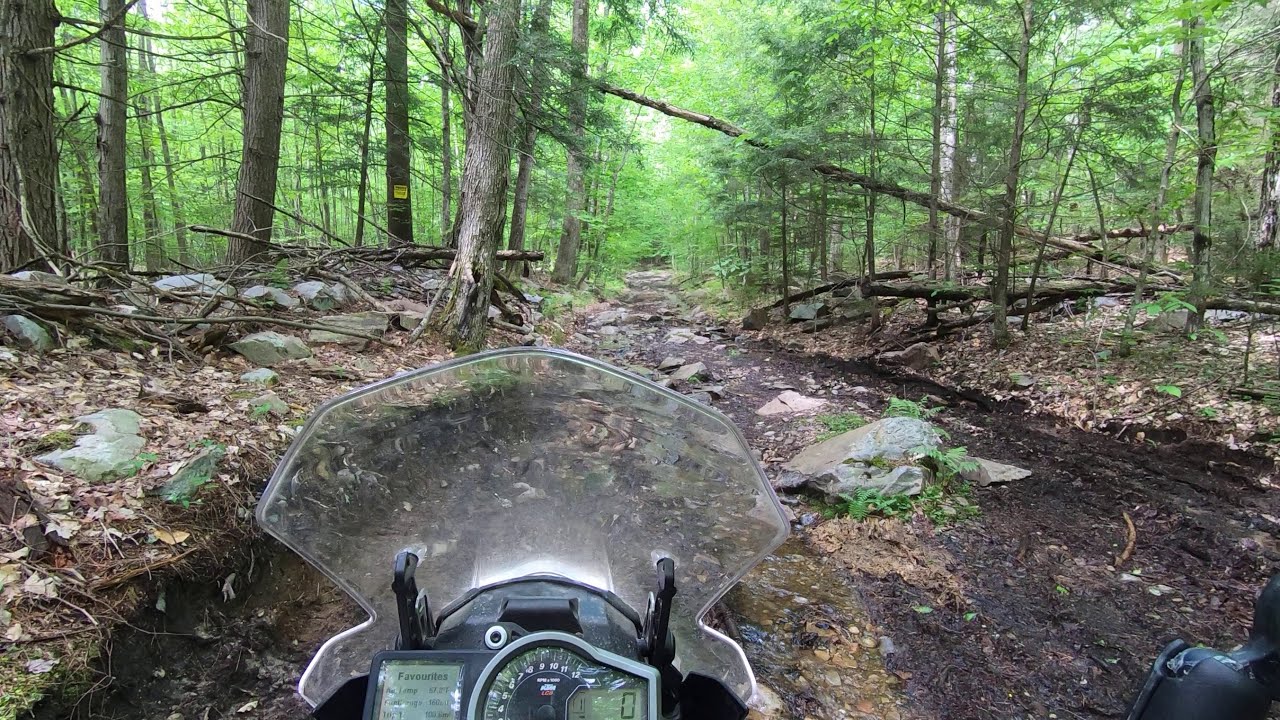This horizontally aligned rectangular picture captures a rugged, wooded area from the vantage point of a stationary off-road motorcycle on a dirt path. Central in the foreground, you can see the bike's dashboard featuring a speedometer reading zero, an electronic display with some text, and a clear plastic windscreen, suggesting the vehicle is a motorcycle rather than a BMX bike. The path itself is dark brown, seemingly moist, and strewn with large rocks, indicating a challenging terrain. Flanked on both sides by tall trees with green leaves, the trail is littered with fallen branches, adding to the roughness of the landscape. A noteworthy feature is a long, narrow branch arching across the path from right to left, hanging high enough for a rider to pass underneath without obstruction. Despite the dense canopy, bits of a bright white sky peek through, signaling it's daytime, likely partly sunny. No people are present in the image, emphasizing the solitude and natural beauty of this forested trail.